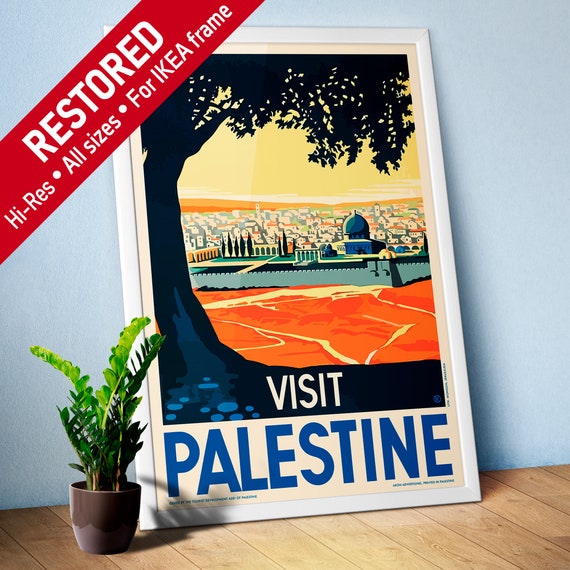The image showcases a vibrant advertisement featuring a framed poster leaned against a light blue wall, resting on a light wooden floor. The poster, encased in a white frame, promotes the beautiful city of Jerusalem with the bold text "Visit Palestine." The artistic illustration on the poster reveals the iconic cityscape of Jerusalem, with notable structures such as the Dome and the surrounding walls. A dark silhouette of a tree with foliage drapes over the city's horizon, complemented by a golden, yellow-orange sky. In the foreground, to the left of the poster, a potted plant with tall, green leaves sits in a brown planter, adding a touch of natural elegance to the setting. A red banner across the upper left corner of the poster reads "Restored, High Res, All Sizes, For IKEA Frame," indicating its compatibility with IKEA frames. Sunlight streams into the room, casting subtle shadows that enhance the overall composition.